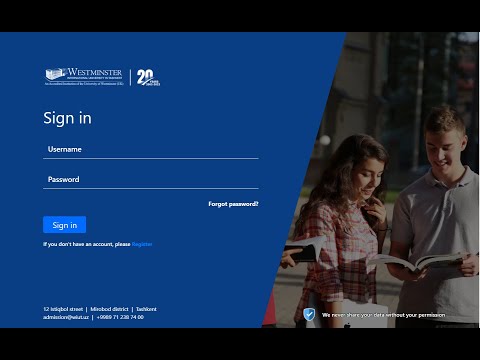This image appears to be a screenshot of a login page from a website. The layout is framed with a black bar at both the top and bottom of the page. The central part of the screen features an angled blue quadrilateral shape. On the right side of this blue section is an image of people reading from a book while standing outside.

At the top of the blue section, there's some unreadable white text, potentially the website's name or slogan. Prominently displayed is what seems to be "Westminster" along with a logo and the number "20." Below this, still in white, are the words "Sign In," followed by labeled fields for "Username" and "Password," each accompanied by an underlining line. To the right of the password field, there's a link named "Forgot Password."

Further down is a medium blue button labeled "Sign In" in white text. Below this button is some additional white text, not fully legible, which includes a blue-colored link, likely for more information or assistance. Underneath, there seems to be more text, possibly containing contact information, though it's not readable.

On the right side, next to the image of people, there is a blue shield icon with more white text.